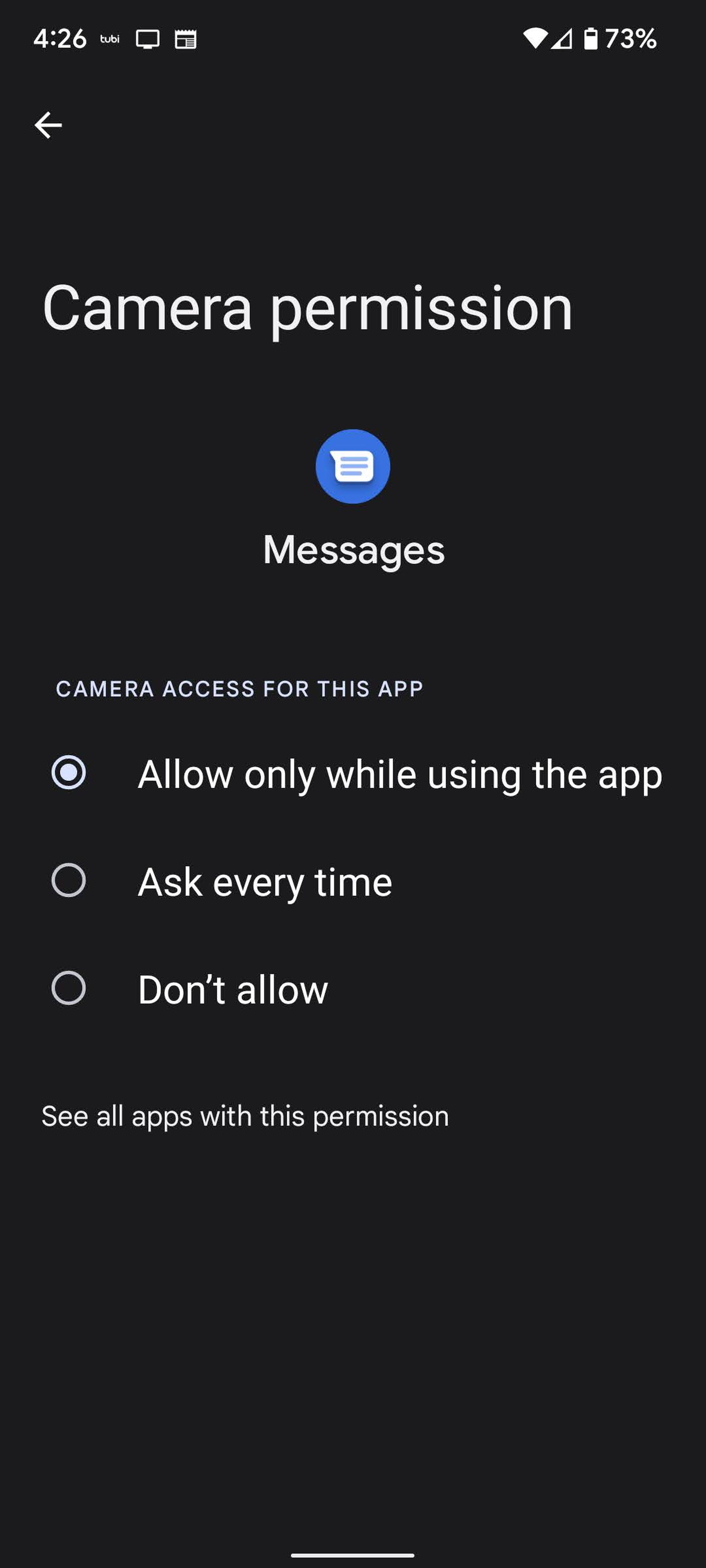The image displays a smartphone screen depicting the camera permission settings. In the top left corner, "426" is prominently shown. Below it, there's a monitor icon next to a news symbol and a WiFi symbol indicating 23% battery remaining.

An left arrow icon precedes the section discussing camera permissions. A blue circle highlights the "Messages" app. The permission status for this app is detailed with a checkmark next to "Allow only while using the app."

Other options are listed but not selected, including "Ask every time" and "Don't allow." Additionally, there's an option to "See all apps with this permission."

The layout includes a black square border around certain elements and a distinct line separating sections. The screen is part of the smartphone's settings interface, specifically showcasing camera access permissions. The overall appearance is very dark, emphasizing the black background.